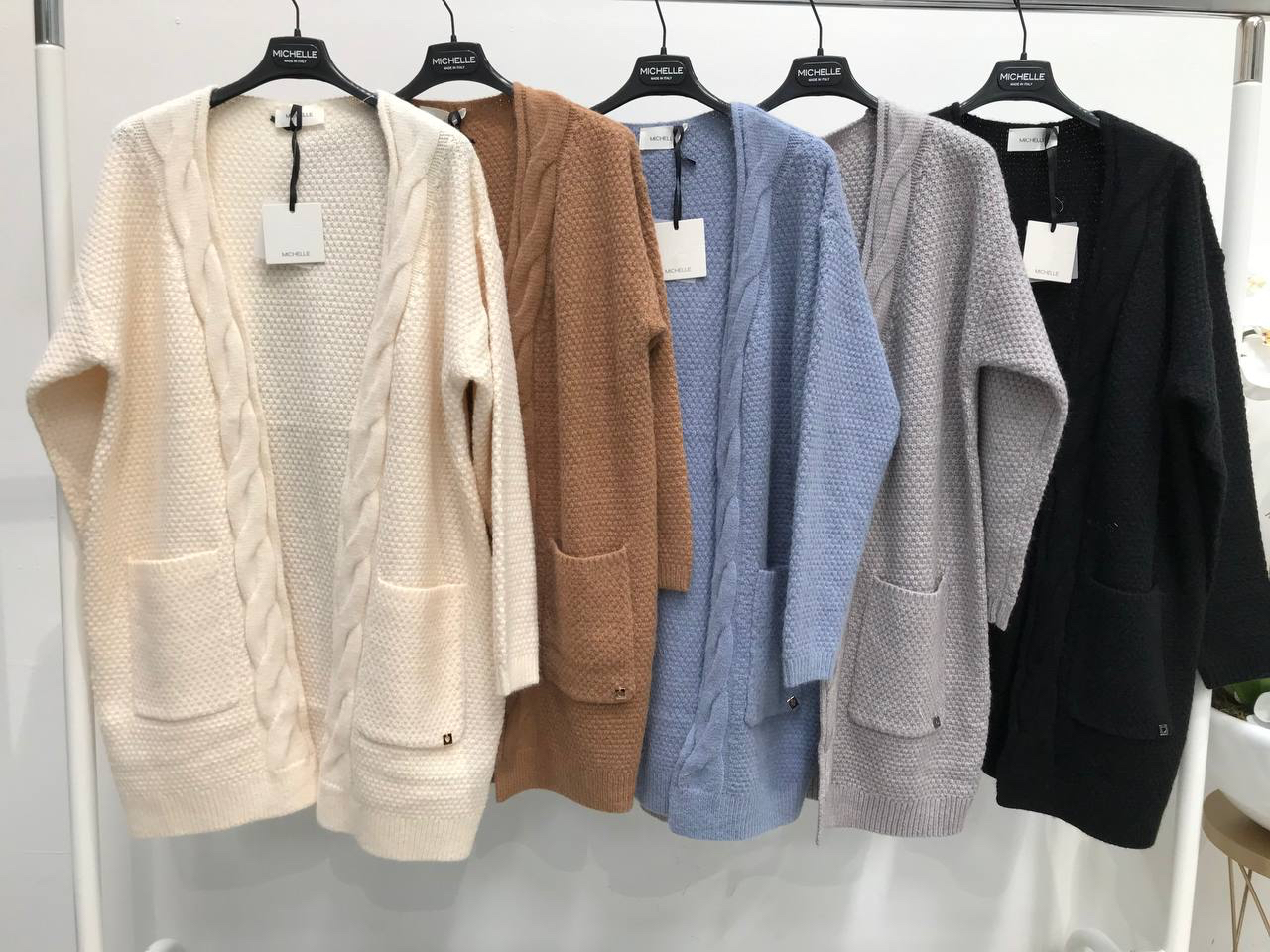This image showcases a detailed display of women's cardigans in a retail shop. The cardigans are arranged on a white rack with a silver rod and white legs, placed against a plain white wall. Each cardigan is hung on a black plastic hanger, all uniformly branded with the name "Michelle" in small white letters. The cardigans, starting from left to right, come in five colors: cream, camel brown, light blue, medium dove gray, and black. Each cardigan features a cable knit design down the front edge, patch pockets on the front, and a ribbed band along the bottom. Hanging from the garment tag at the back of each neck is a white hang tag attached by a piece of black ribbon, displaying product details and pricing. Additional background details include a hint of a small table with a stool and a white sheet casting shadows, lending a casual retail ambiance to the scene.